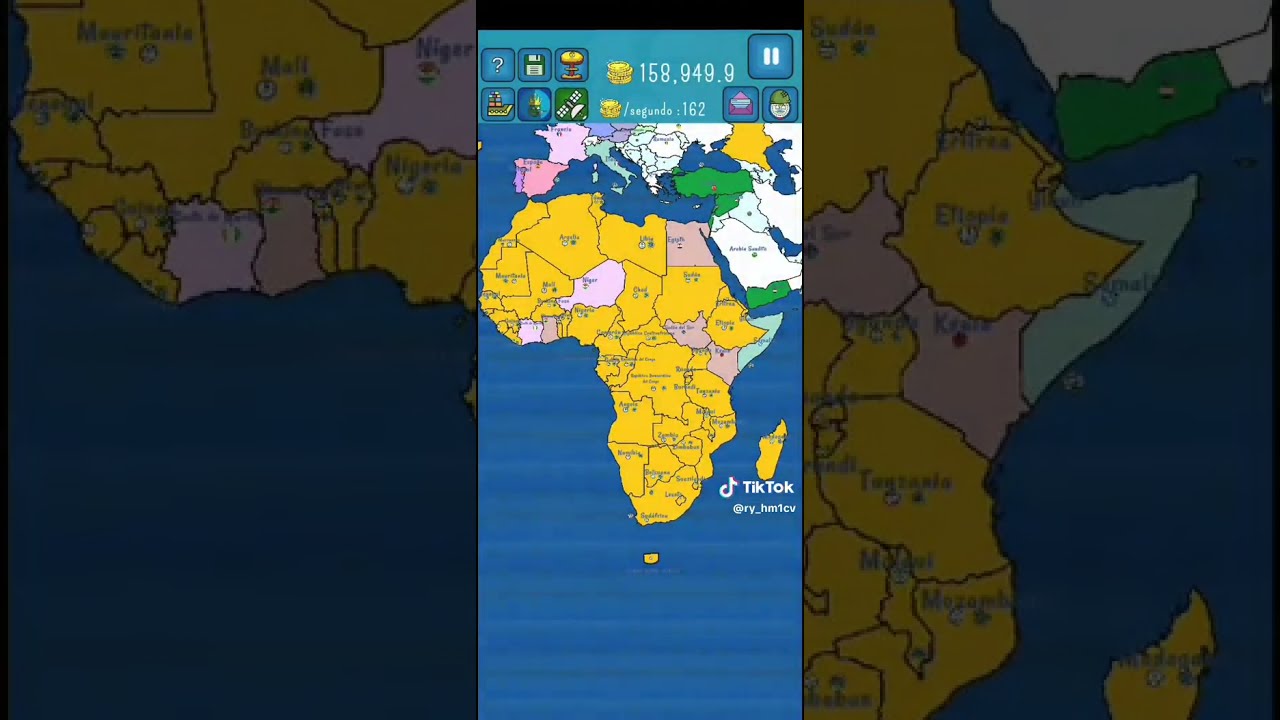The image is a detailed screenshot from a game displayed on TikTok, featuring a map of Africa predominantly in a mustard yellow color, with various countries outlined and separated by distinct lines. Surrounding Africa, the map also shows parts of Europe, the Middle East, and Asia, with countries in diverse hues such as pink, dull purple, light blue, white, green, and orange. The dark blue ocean serves as the background, accentuating the landmasses. At the top of the image, game icons include a pause button, an envelope, an army soldier, a save icon, a mushroom cloud indicating a nuclear explosion, an airplane, a ship, and a question mark for more information. Additionally, a TikTok logo and a user’s account name are prominently displayed at the bottom right of the image, suggesting that this is a screenshot from a player’s game shared on the social media platform. Superimposed on the map is a smaller, vertical rectangle showing the same content on a smaller scale but in brighter colors, which also expands to include parts of Europe and the Middle East.